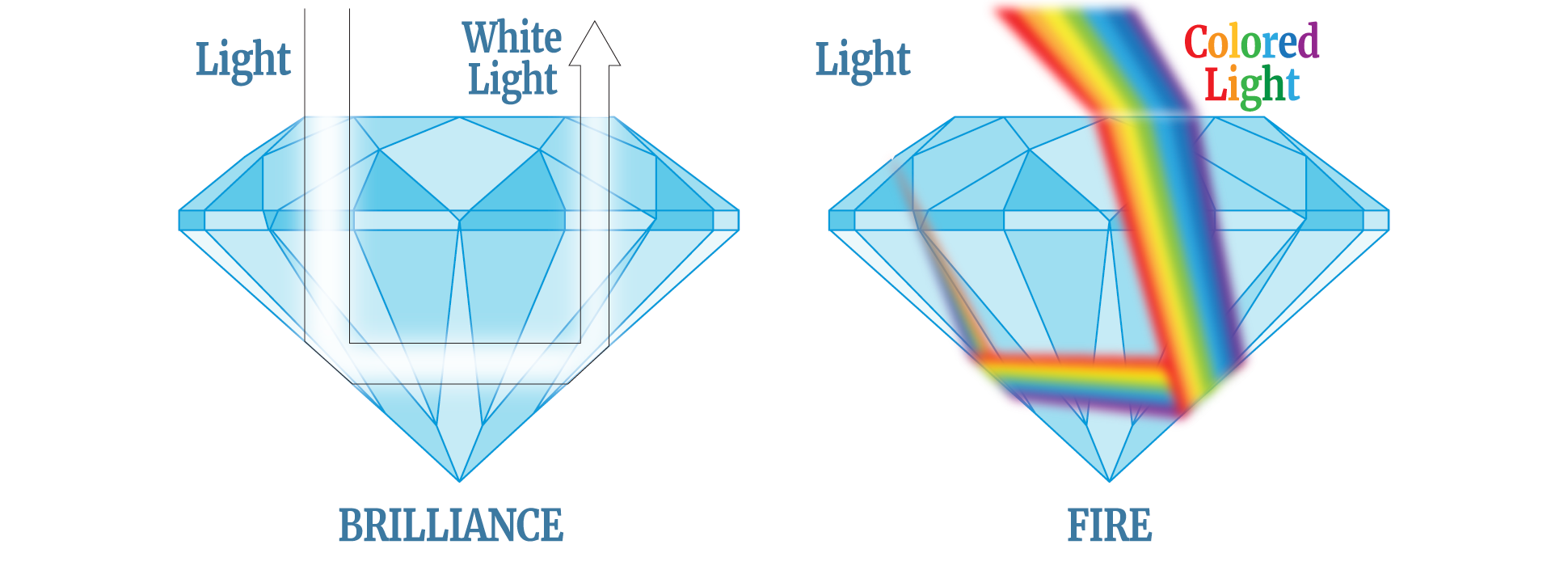This detailed diagram illustrates how light behaves when it enters a diamond, emphasizing the differing outcomes of brilliance and fire. The image displays two diamond shapes side by side, both depicted with varying shades of blue. The left diamond is labeled with "light" at the top, "brilliance" at the bottom, and "white light" near a path indicated by a thick white arrow with a black outline, which travels downward, then to the right, and finally upwards. The right diamond follows a similar structure but is marked with "light" at the top, "fire" at the bottom, and "colored light" along a rainbow-colored path that moves downward, then upward, and out, symbolizing the dispersion of light into various colors. This rainbow gradient includes red, orange, yellow, green, blue, and purple hues, showcasing how light splits to create the effect known as fire. The overall effect captures how white light results in brilliance and colored light results in fire when interacting with the facets of a diamond.